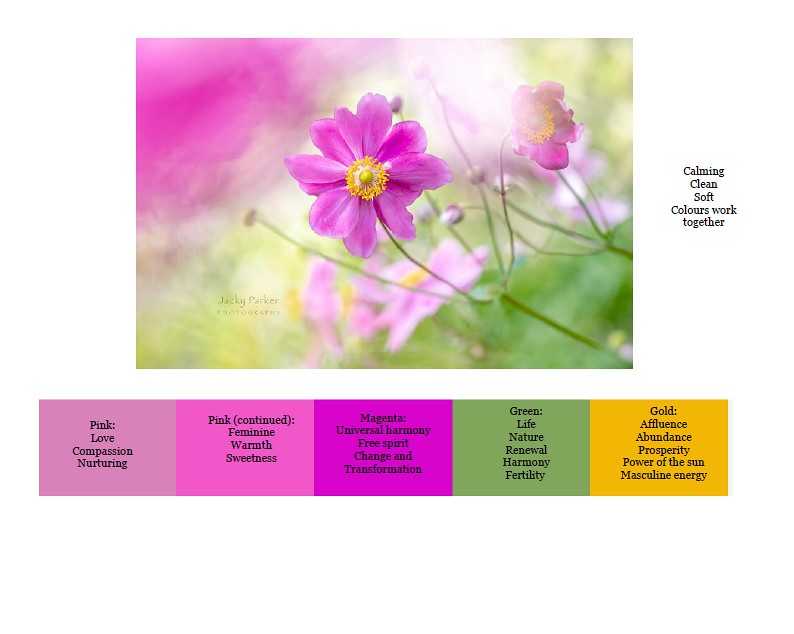The image showcases a pair of striking lavender purple flowers in full bloom, each with delicate petals encircling a central ring of golden pollen that subtly transitions into a creamy white. Nestled amid lush green foliage, the flowers appear vibrant and fresh, as if photographed in a serene countryside garden. The photograph, credited to Jackie Parker as noted in faint text, exudes a calming and clean aesthetic. Accompanying the image on the right is a set of descriptive words emphasizing the soft colors and their harmonious qualities. Below, multiple colored boxes display the associated text in black, detailing the characteristics of each color: pink (love, compassion, nurturing; feminine, warmth, sweetness), magenta (universal harmony, free spirit, change, and transformation), green (life, nature, renewal, harmony, fertility), and gold (affluence, abundance, prosperity, power of the sun, masculine energy). The artwork provides a detailed and enriching visual experience, accentuated by the thoughtful interplay of color and meaning.